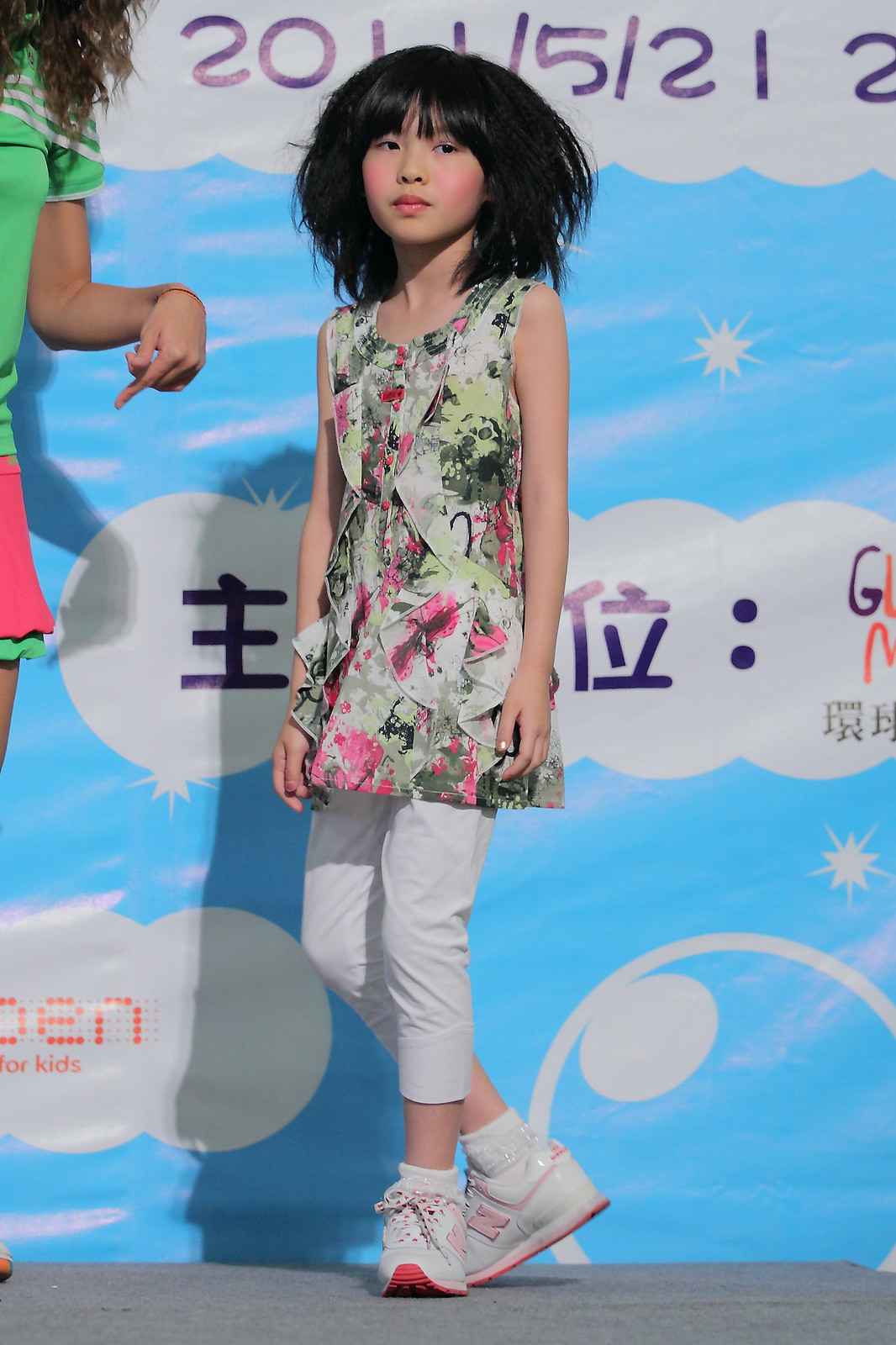This image depicts an Asian girl, likely younger, standing on a stage or in front of an advertisement with a background that features a blue sky with puffy white clouds, white stars, and curved lines. Her hair is shoulder-length, black, and quite frizzy. She is wearing makeup, noticeable with red cheeks, and a multicolored, sleeveless floral top that extends down to her fingertips, nearly reaching her thighs. She pairs this with white capri pants, white socks, and white tennis shoes which have a distinctive pink "N" on the side. Her arms are relaxed and by her sides, and she’s glancing out of the left side of her eyes.

To the left of the girl, partially visible, is another taller female who seems to be dressed in a green top and a pink dress skirt; she is pointing downward with her index finger. The stage or surface they stand on is gray. Additionally, the setting is likely indoors, possibly at a seminar, conference, or school event. The scene is somewhat obscured by inscrutable black text in another language against the blue and white background, further emphasizing the girl as the focal point of the image.